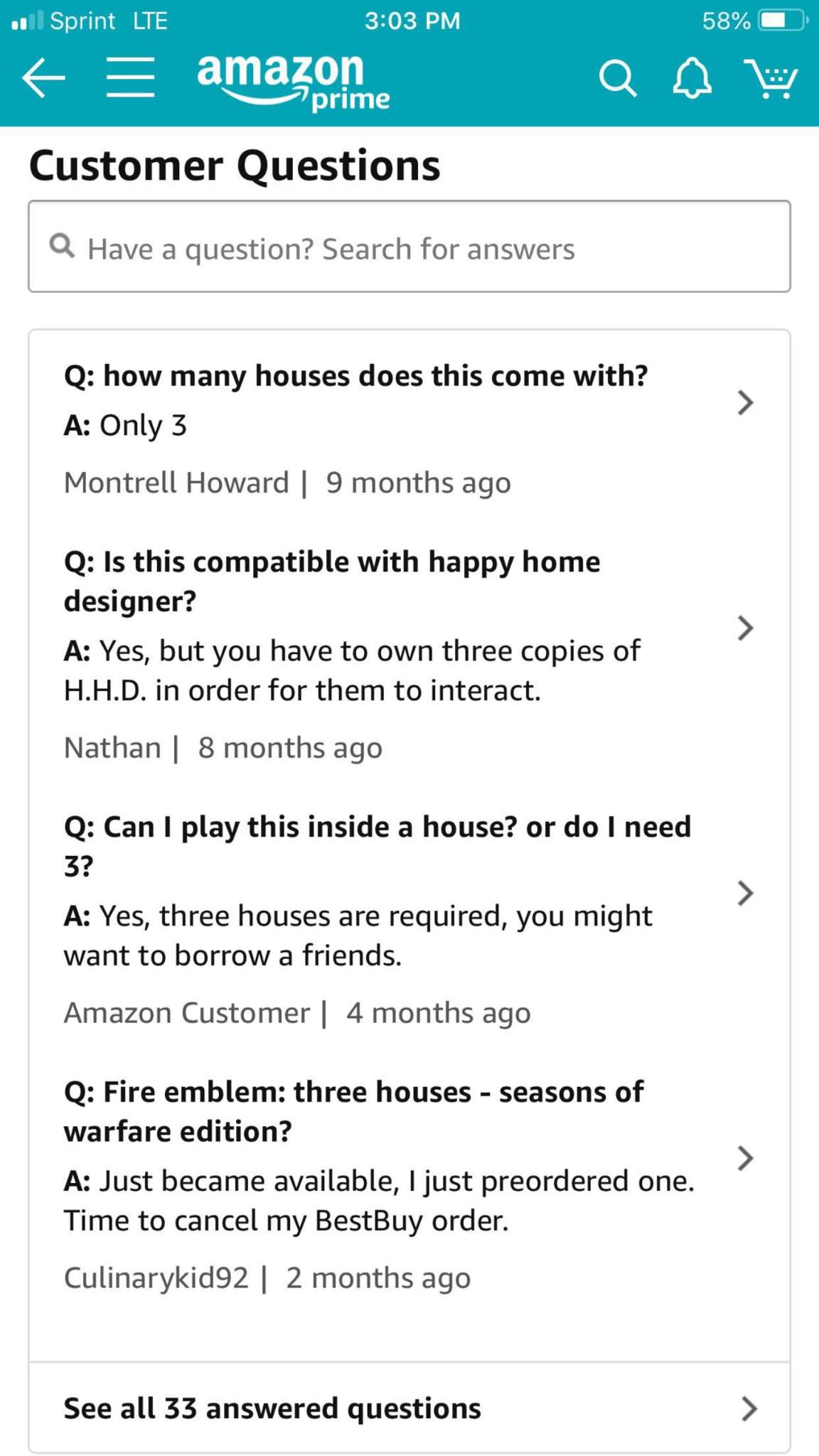A detailed screenshot of the Amazon Prime app displayed on a cell phone. The screen shows the "Customer Questions" section with the Sprint LTE network, two bars of signal strength, and the time indicated as 3:03 PM in the top left corner. The battery meter displays 50% charge. At the top left of the interface, features such as a back arrow and a hamburger menu are present. The header reads "Amazon Prime" in white text, situated on a light teal background. On the top right, you'll find icons for search (magnifying glass), notifications (bell icon), and the shopping cart, all in white.

Below this header, the title "Customer Questions" is bold and black, with a search field underneath where users can type "Have a question? Search for answers." The screen shows four sample questions with their respective answers.

1. **Q: How many houses does this come with?**
   **A: Only three.** - Montrell Howard, nine months ago.

2. **Q: What is compatible with Happy Home Designer? Is this compatible?**
   **A: Yes, but you have to own three copies of HHD in order to interact.** - Nathan, eight months ago.

3. **Q: Can I play this inside a house, or do I need three?**
   **A: Yes, three houses required. You might want to borrow a friend’s.** - Amazon Customer, four months ago.

4. **Q: Fire Emblem, Three Houses, Seasonal Warfare Edition.**
   **A: Just became available. I preferred one. Time to cancel my Best Buy order.** - Culinary Kid 92, two months ago.

At the bottom, there is a "See all 33 answered questions" option, also bold, with a gray right-facing arrow next to each question, answer, and the "See all" link, indicating that users can click to see more information.